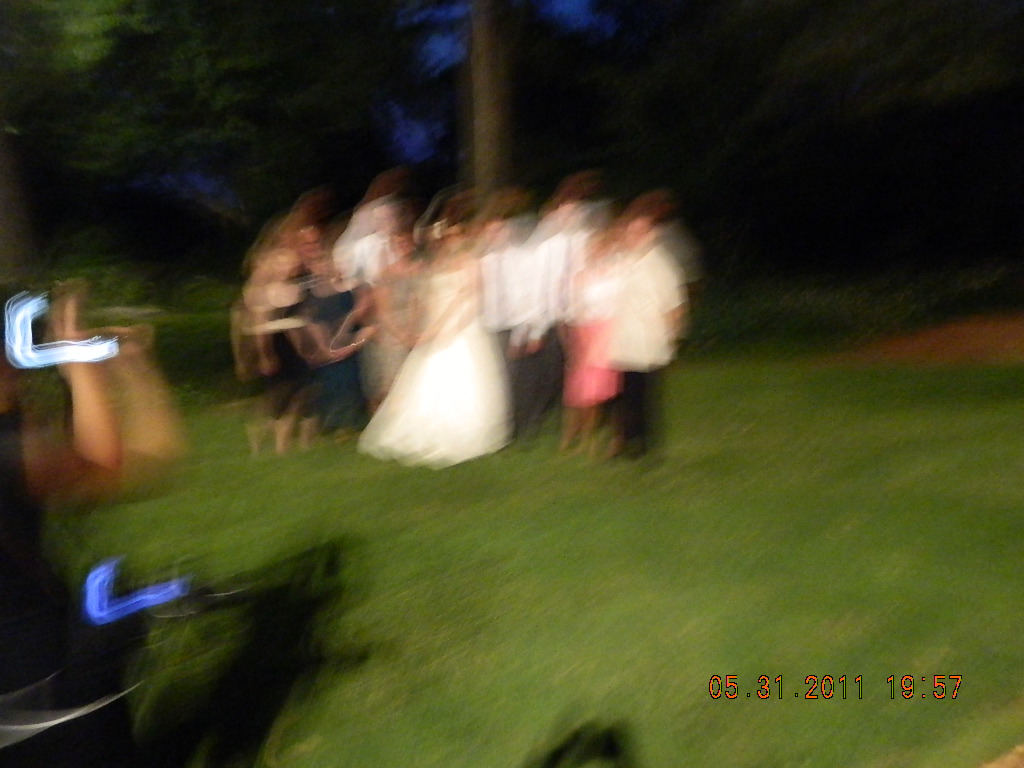This image captures a very blurry and dimly-lit outdoor wedding scene at nighttime. Illuminated by a bright white light, shadows of people are visible on the ground to the left and center. In the middle of the photograph stands a bride in an off-the-shoulder, flowing white wedding gown, surrounded by multiple people. To her right, several men are dressed in white shirts, some with ties and dark pants. Among them, one man is notably wearing a white shirt without a tie. Beside the bride on either side, women are adorned in dresses of various colors, including two in elegant black evening wear and one in a white top with a pink skirt. Further to the left, the figures become less distinct, but it is evident they are also in formal attire. The group is posing on a grassy lawn, and behind them rises a large wooden pole and the trunk of a tree. The photographer's hand is faintly visible to the left side, and a time stamp reading "05.31.2011, 19:57" is embedded in the lower right corner of the photo.